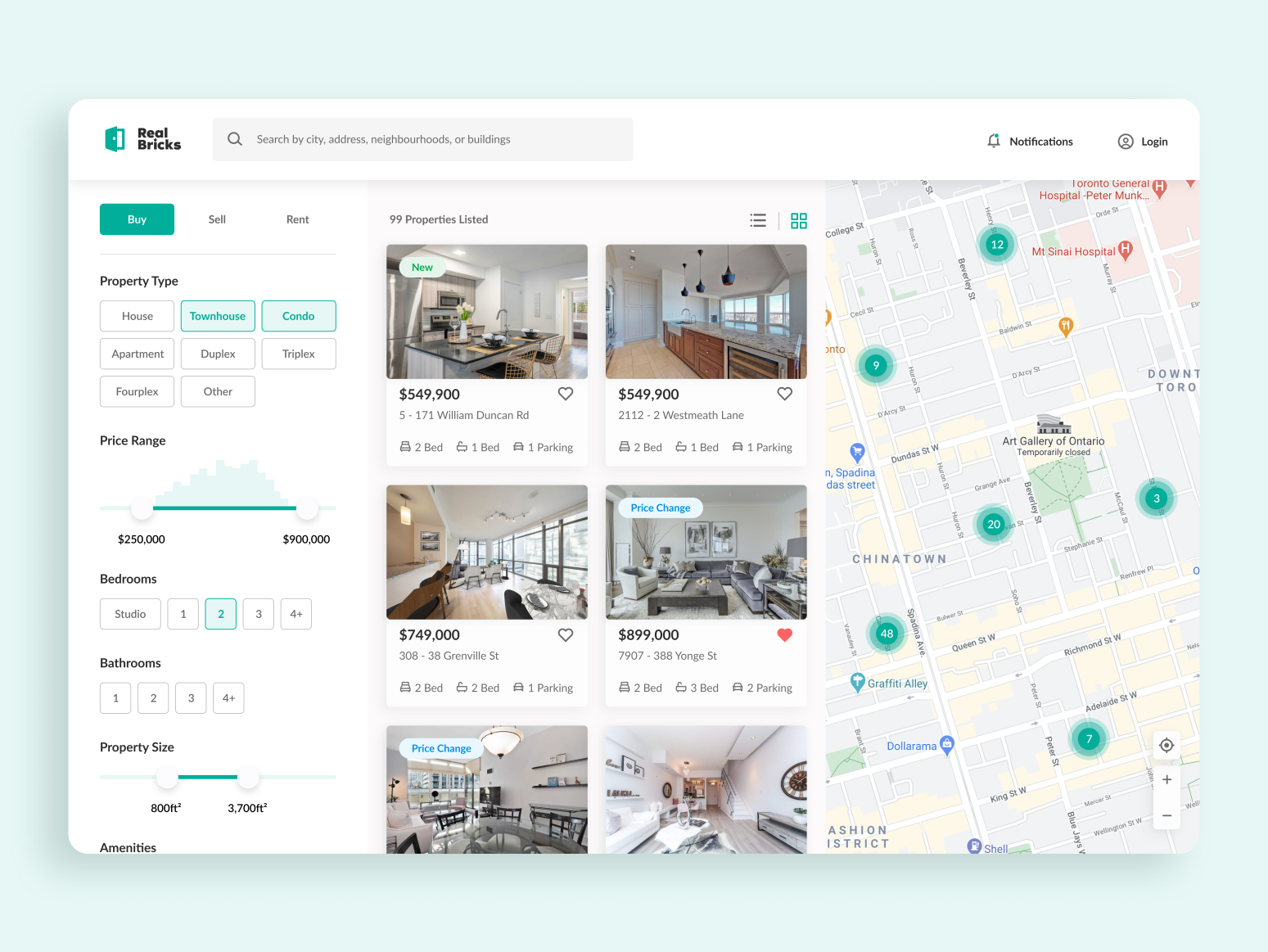**Detailed Caption:**

This is a detailed screenshot from the real estate website, Real Bricks, featuring a user-friendly interface designed for property seekers. The brand’s logo is prominently displayed, showing a slightly open door icon in a shade of blue or dark green. Adjacent to the logo is a comprehensive search box, and on the far right of the same row, there are icons for notifications (shaped like a bell) and user login.

The homepage is split into distinct sections, with a map on the right, pinpointing various properties around New York’s Chinatown. To the left is a filter pane that allows users to refine their search criteria. The filter options include tabs for 'Buy', 'Sell', and 'Rent', along with property types such as 'Houses', 'Townhouses', and 'Condos'. Currently, the 'House' and 'Condo' filters are highlighted in green.

Property specifications are detailed with a price range slider set between $250,000 and $900,000. Bedroom options vary from studios to properties with four or more bedrooms, with the '2 bedrooms' filter highlighted. Bathroom options range from one to four. The property size filter is set between 800 square feet and 3,700 square feet. 

The website lists 99 properties, each accompanied by a thumbnail image. Eight properties are showcased here. The first in the list is a modernly designed kitchen area for a condo priced at $549,900, featuring 2 bedrooms, 1 bathroom, and 1 parking space, marked as 'New'. 

Next to it is another condo with wide picture windows, also priced at $549,900, offering 2 bedrooms, 1 bathroom, and 1 parking space, with the specific address provided. 

Further down is a photo of a contemporary living room featuring a sectional sofa and a black flat coffee table, listed at $899,000. This listing has a red 'favorite' heart icon marked, indicating it has been saved by a user, along with a 'price change' tag. It offers 2 bedrooms, 3 bathrooms, and 2 parking spaces.